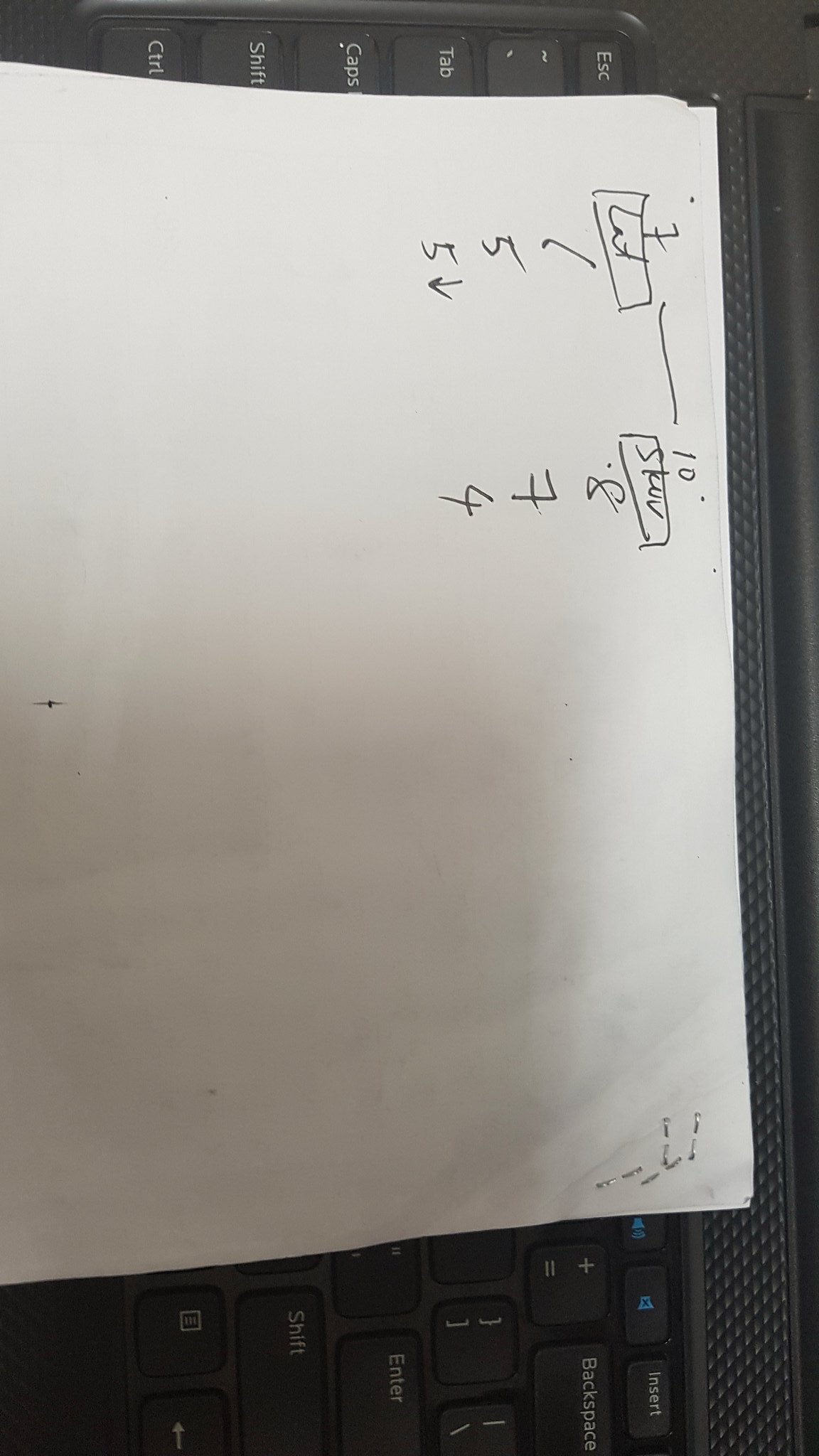This photograph features a black keyboard positioned vertically, rotated 90 degrees so the left side is at the top and the right side at the bottom. Resting on the keyboard is a piece of white paper. In its current orientation, the bottom right corner of the photo corresponds to the top right corner of the paper itself, where the backs of four staples are visible, binding together at least two sheets.

In the top left corner of the paper (which appears at the top right in the rotated photo), a hand-drawn table is present. The first row of the table lists the number "7" followed by the letters "LAT," marked in ink or heavy pencil within a rectangle. Below this, there appears to be a sequence starting with "1," followed by "5" twice, and a downward arrow. Further to the right within this table, at the top, the number "10" is written next to "SKU" (possibly abbreviated), which is checked off and enclosed within another rectangle. Below these, the numbers "8," "7," and "4" are listed sequentially.